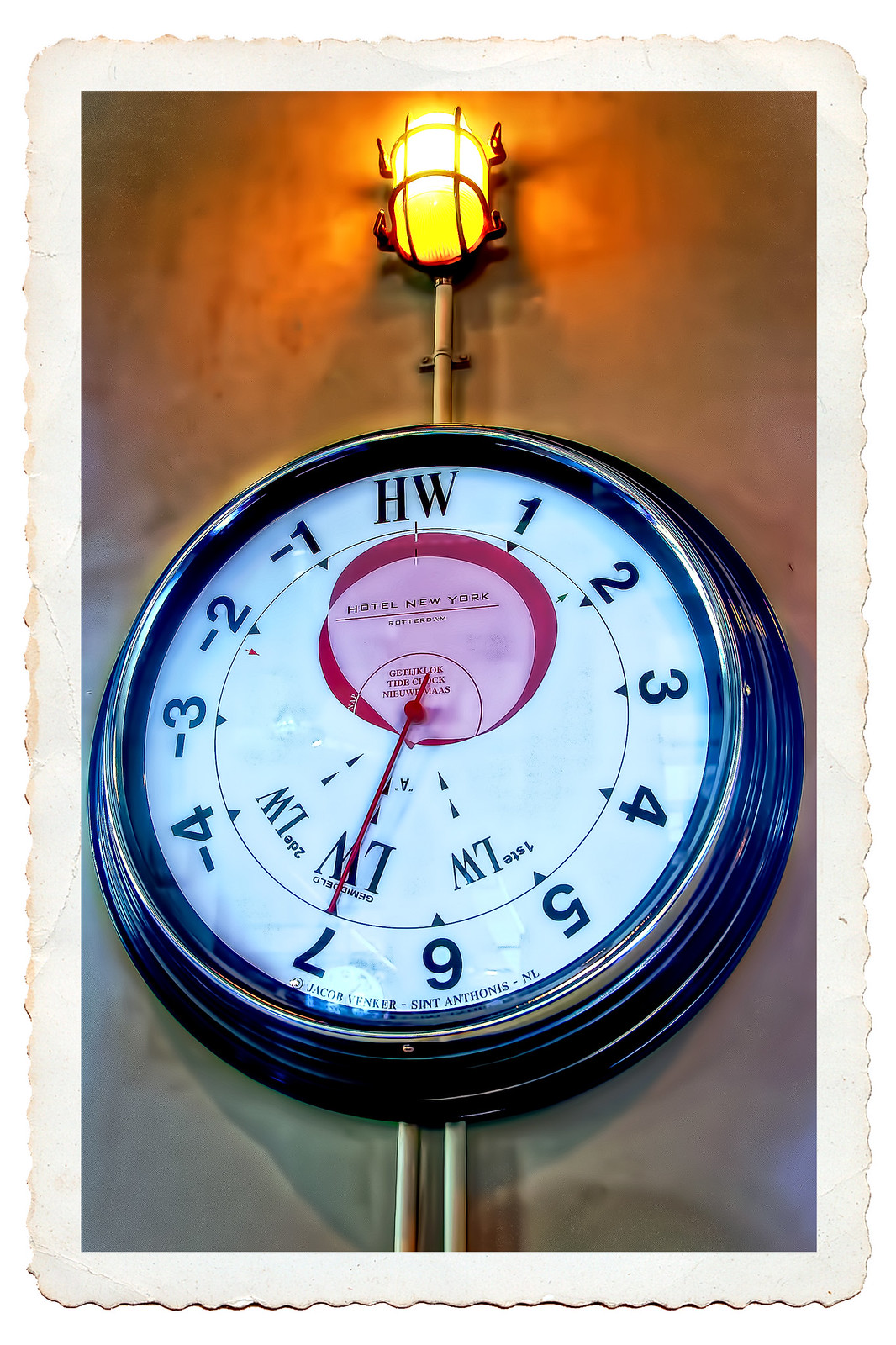This image showcases a unique wall clock mounted against a wood-colored backdrop. The clock features a black border and a distinct face void of any white areas. A yellow light with a wire cage protrudes from the top of the clock, adding an industrial flair. Highlighted at the top of the clock face is an inscription "HW."

The numbering on the clock face is unconventional, displaying a sequence that reads: "1, 2, 3, 4, 5, 6, 7", followed by "minus 4, minus 3, minus 2, minus 1." At the lower portion around the 6 and 7 positions, it repeats "LW LW LW" in an upside-down manner. There is a small red circle near the top, inscribed with "New York." Interestingly, the hour, minute, and second hands all converge and point directly at the number 7. This clock combines quirky design elements with an artistic twist, creating an eye-catching and thought-provoking piece.